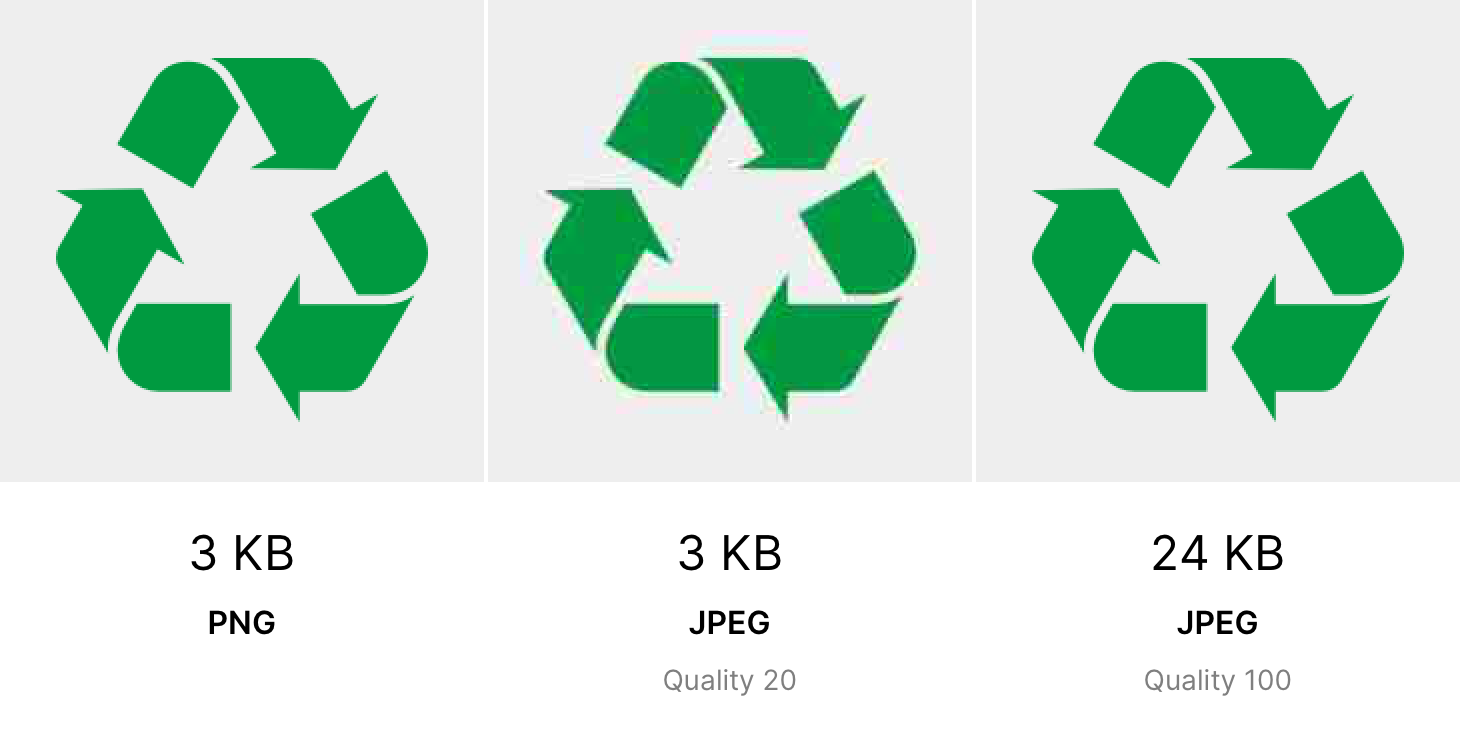The image depicts three side-by-side recycling symbols, each featuring three green arrows forming a triangular shape synonymous with recycling. All symbols are placed on individual gray backgrounds. Below each symbol, there are text labels detailing their file characteristics and quality. The first symbol, on the left, is labeled "3 KB PNG" and appears clear. The middle symbol has the label "3 KB JPEG, quality 20," indicating it is of lower quality with noticeable blurriness and artifacts. The third symbol, situated on the right, is labeled "24 KB JPEG, quality 100," and is the clearest and highest quality image among the three. The text beneath the images is predominantly in black against a white background, with some variations in gray, emphasizing the differences in file type, size, and quality.